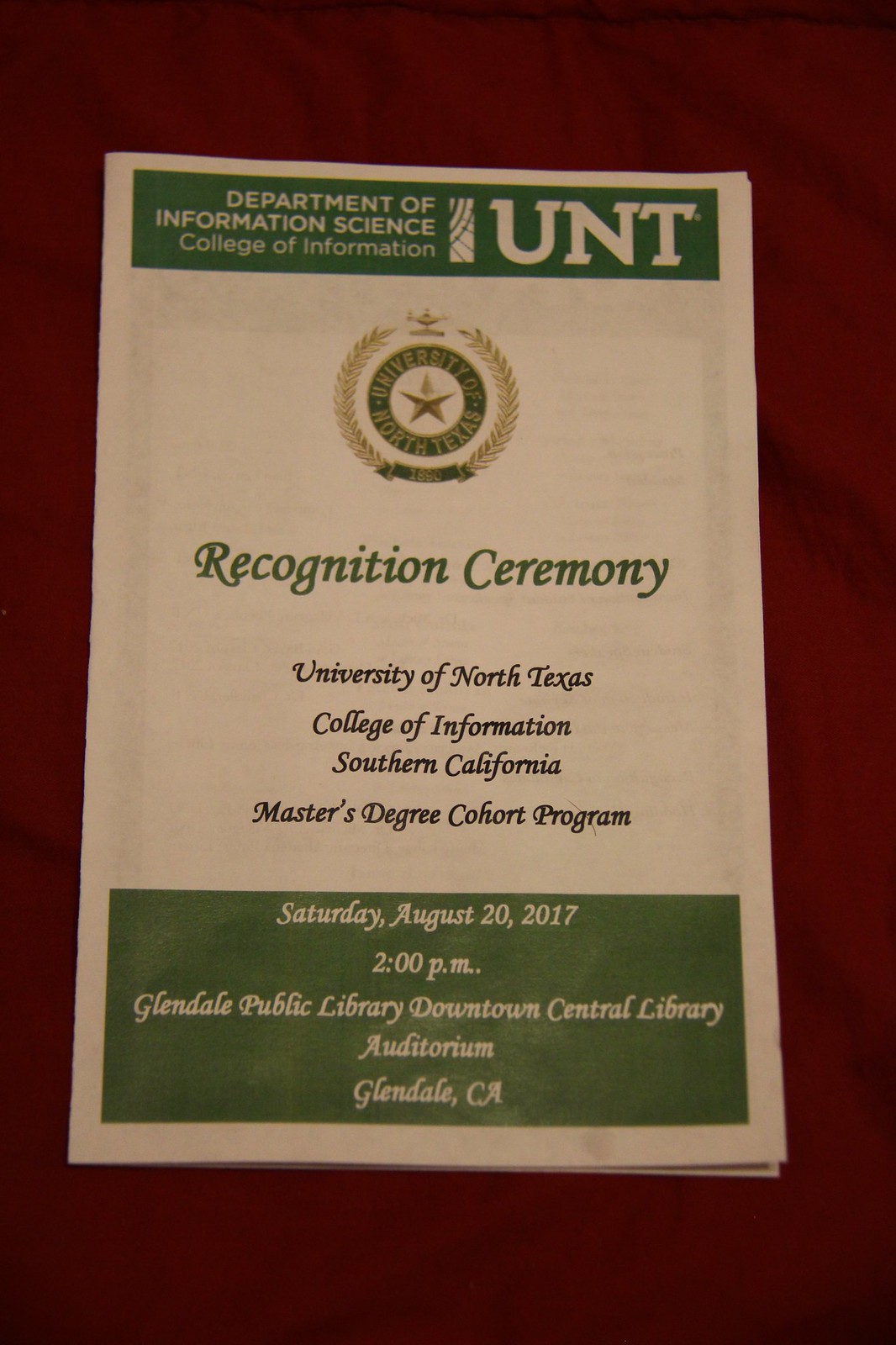This image features a detailed photograph of a green and white brochure, prominently displayed against a textured red surface, possibly a table or fabric. The brochure is meant for a recognition ceremony organized by the University of North Texas (UNT). The top part of the brochure showcases a green background with white text that reads "Department of Information Science, College of Information, UNT," alongside a stylized emblem with a star and wheat design. Below this in green cursive text lies the phrase "Recognition Ceremony," followed by "University of North Texas, College of Information, Southern California, Master's Degree Cohort Program" in black text. Toward the bottom, another green section provides event details in white: "Saturday, August 20th, 2017, 2 p.m., Glendale Public Library, Downtown Central Library, Auditorium, Glendale, California." The brochure appears to be multi-paged and possibly stapled along the side.